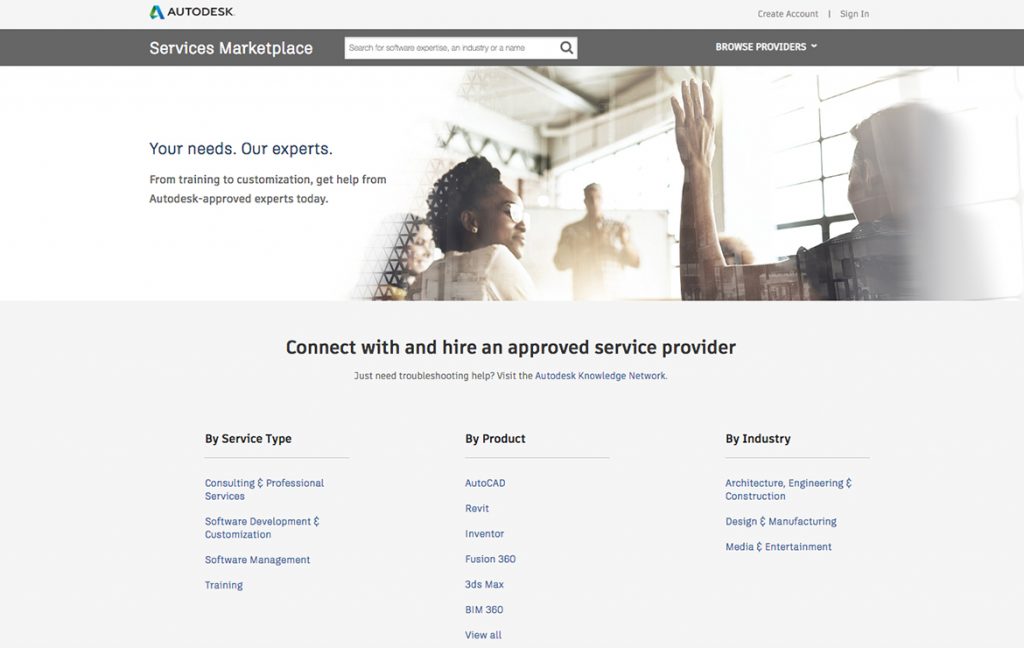This detailed caption accurately describes the elements of the image, organizing the information into a clear and structured format:

---

At the top of the image is a thin header with a light gray background. On the left side of this header, there is a teal logo resembling a stylized paper "A". To the right of the logo, in dark gray capital letters, is the text "Autodesk," likely followed by a period.

Below this header is a thin strip of medium gray. On the left side of this strip, the text "Service Marketplace" is displayed in white. Towards the right, there is a rectangular search bar with a white background. Inside the search bar, in gray text, it says "Search for Software Expertise, an industry, or a name." To the right of this text is a dark gray magnifying glass icon. Further to the right, in white capital letters, is the text "Browse Providers," accompanied by a downwards-pointing arrowhead to indicate a submenu.

Following this strip is a banner. On the right side of the banner, a woman is depicted with her left hand raised. To her left, there's another woman wearing glasses and a white shirt, looking directly at the first woman. In the background, a man is seen at the far back center.

On the left side of the banner, in navy text, is the phrase "Your Needs. Our Experts." Below this in smaller black font is the text "From training to customization, get help from Autodesk-approved experts today."

Beneath the banner is a rectangular area with a light gray background. At the center of this area, in black text, is the message "Connect with and hire an approved service provider." Underneath this, in smaller black text, is the question "Just need troubleshooting help?" followed by the clickable blue text "Autodesk Knowledge Network."

Three headers are listed in bold black text near the bottom: "By Service Type," "By Product," and "By Industry."

---

This detailed caption provides a comprehensive and precise description of the image, clearly conveying the visual layout and content.